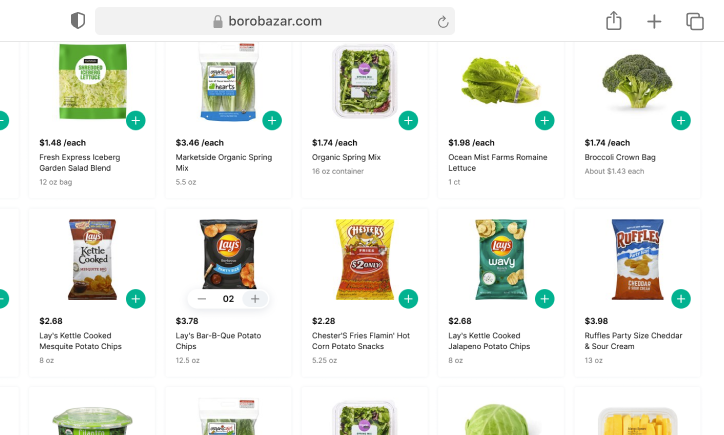The image is a screenshot from the shopping website borobazaar.com, featuring a selection of grocery items displayed against a white background. At the top of the screenshot, there are various icons including a shield icon on the left and plus, copy, and upload icons on the right.

The image shows two and a half rows of products, although the bottom row is partially visible. Each product has a description, price, and in some cases, weight details.

- **Top Left Corner:**
  - A green bag labeled "Fresh Express Iceberg Garden Salad Blend" priced at $1.48 each, containing 12 ounces of lettuce.

- **Following Products:**
  - "Marketside Organic Spring Mix," priced at $3.46 each for 5.5 ounces of thin salad leaves.
  - Another "Organic Spring Mix," priced at $1.74 each for an 18-ounce container of salad leaves.
  - "Ocean Mist Farm Romaine Lettuce," priced at $1.98 each for an unspecified weight, likely without packaging.

- **Next Row:**
  - A bag of broccoli crowns priced at $1.74 each, containing one head of broccoli.
  - A bag of "Lays Kettle Cooked Mesquite Potato Chips," priced at $2.88 for 8 ounces.
  - A bag of "Lays Barbecue Potato Chips," priced at $3.78 for 12.5 ounces.
  - "Chester's Fries Flamin' Hot Corn Potato Snacks," priced at $2.28 for a 5.25-ounce bag.
  - "Lays Kettle Cooked Jalapeno Potato Chips," priced at $2.68 for an 8-ounce bag.
  - "Ruffles Party Size Cheddar and Sour Cream Chips," priced at $3.98 for a 13-ounce bag.

To the right of each product, there are plus icons, presumably for adding items to the shopping cart.